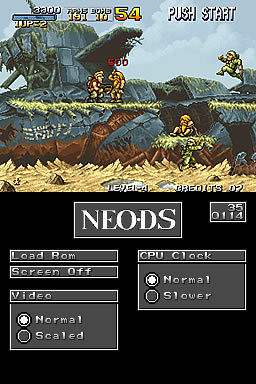The image depicts a screenshot from an emulated arcade game, specifically "Metal Slug," running on a smartphone in portrait mode, characteristic of the narrower and taller aspect ratio of mobile screens. The top half of the image showcases the detailed, mechanized digital artwork of the game, where a player is seen rescuing a civilian while another civilian is approached by a soldier. In the midst of the action, a red "500" hovers above the characters, indicating a score or damage tally. Prominently displayed in the upper right-hand corner is the prompt "PUSH START" in white capital letters, alongside a large, yellow-to-orange gradient number "54." The game screen is filled with visual elements like grass and elevated platforms, creating a dynamic environment for combat.

The bottom half of the image transitions to a black background featuring several functional rectangles arranged in a utilitarian layout typical of emulator interfaces. At the top of this section, we see "NEO.DS" or "NEODS," identifying the emulator being used. Below this, on the left side, slim rectangular boxes are labeled "LOAD ROM" and "SCREEN OFF," respectively. Further down is a wider rectangle marked "VIDEO," with selectable options “NORMAL” and “SCALED,” indicated by dots where the top option is highlighted. To the right, another similar-sized rectangle titled "CPU CLOCK" presents the options “NORMAL” and “SLOWER,” again with dots for selection indication. Numbers "35" and "0114" are displayed in smaller boxes, likely representing arcade tokens or operational metrics of the emulator. The intricate emulator interface overlays further illustrate the detailed setup for playing this classic arcade game on a modern smartphone device.